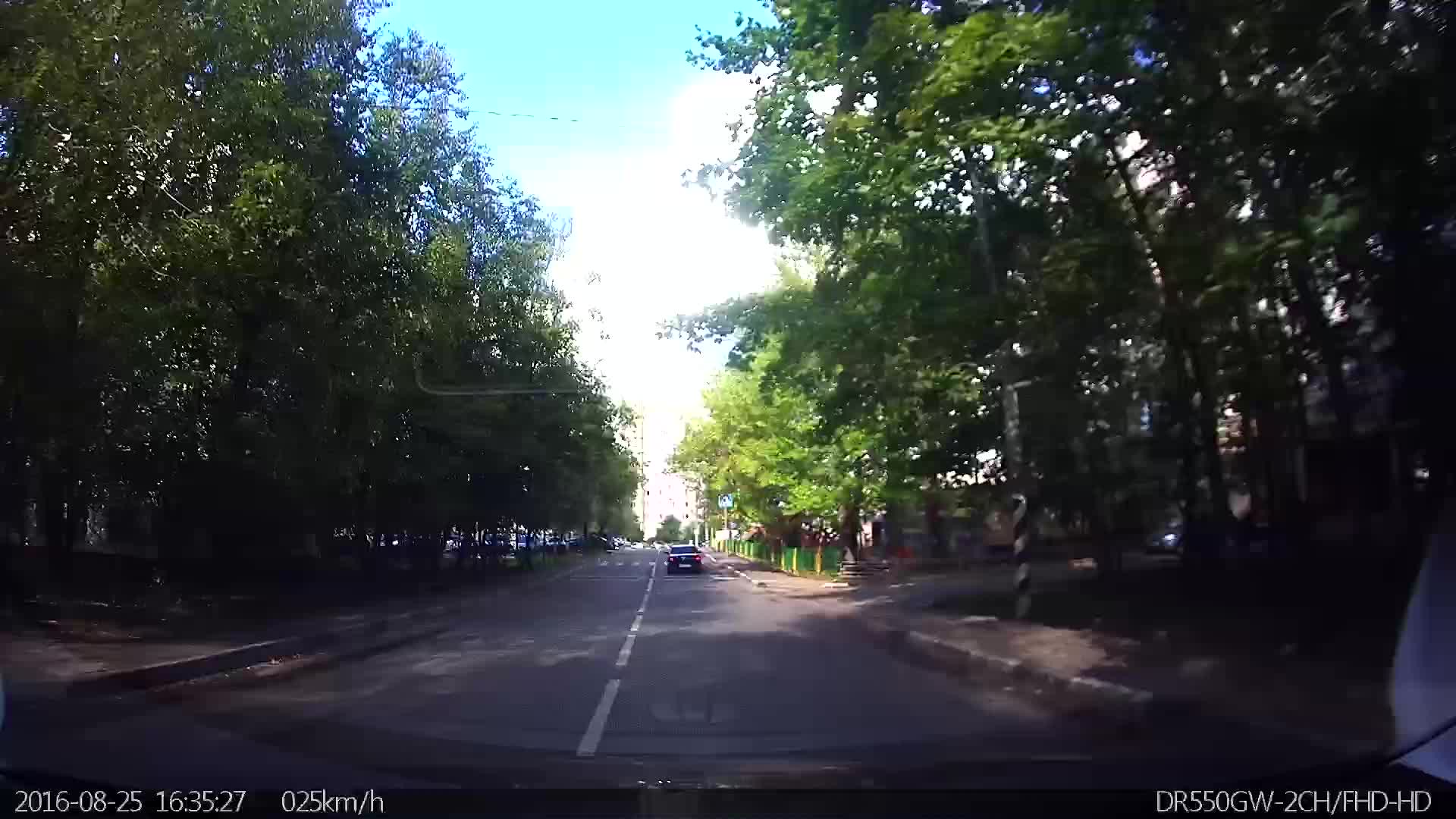Captured from a dashcam, this image reveals a straightforward stretch of road bordered by lush greenery on both sides, characteristic of a serene yet slightly remote area. Central to the frame, a car is seen traveling ahead, maintaining a position slightly to the left. Surrounding the road, verdant trees line both sides beyond the sidewalks, creating a canopy of foliage that adds a touch of natural beauty. At the bottom of the image, embedded data indicates the exact moment of capture: "2016-08-25, 16:35:27," and records the vehicle's speed at 25 kilometers per hour. The bottom right corner of the image displays the camera model used: "DR550GW-2CH-FHD-HD."